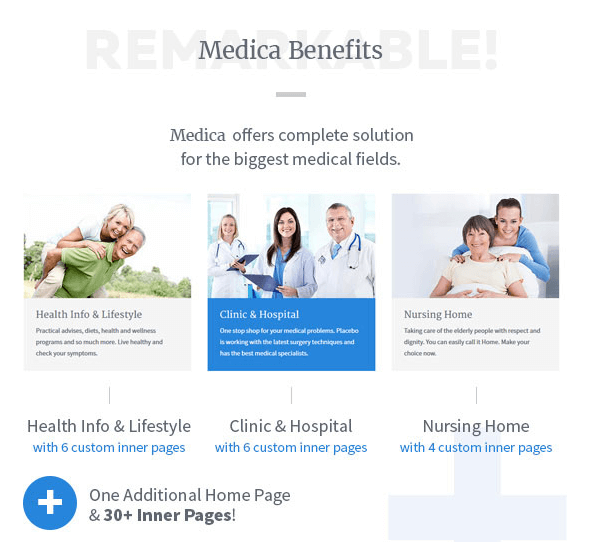The image showcases a triptych layout on a medical-themed information page. Centered at the top, the header reads "Medica Benefits" in a bold gray font against a white background. Overlaying this in a translucent, bold font is the word "Remarkable!" emphasizing the impressive nature of the services offered.

Beneath this header, a subtitle declares, "Medica offers complete solutions for the biggest medical fields," setting the stage for what follows.

The lower section is divided into three distinct images, each accompanied by informative text:

1. The left image features a woman in a white shirt giving a piggyback ride to a man in a green shirt. The surrounding text reads, "Health Info and Lifestyle: Practical Advice, Diets, Health and Wellness Programs, and so much more. Live healthy and check your symptoms." This highlights the lifestyle and informative aspect of the services provided.
   
2. The central image, set against a blue background, shows three people dressed in white lab coats. The text above them reads, "Clinic and Hospital: One Stop Shop for Medical Problems. Placebo is working with the latest surgery techniques and has the best medical specialists." This section emphasizes the cutting-edge medical care and expertise offered by Medica.

3. The right image depicts a woman in a tan shirt with another woman in a long-sleeved blue shirt. The associated text explains, "Nursing Home: Take care of elderly people with respect and dignity. You can easily call it home. Make your choice now." This highlights the compassionate and respectful care available for the elderly.

At the bottom of the page, additional text details the organizational structure and navigation options available: "Health Info and Lifestyle with six custom interpages, Clinic and Hospital with six custom interpages, Nursing Home with four custom interpages, and one additional home page with 30+ interpages." This underscores the extensive and user-friendly resources provided by the Medica platform.